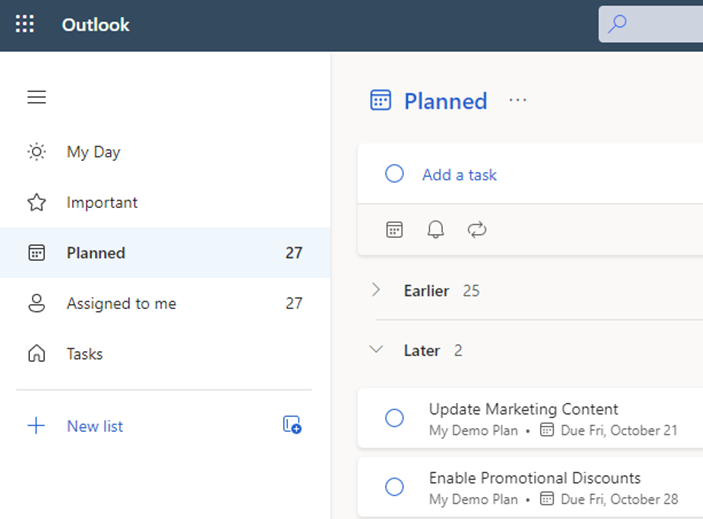This screenshot showcases the interface of Microsoft Outlook's mail program. The top of the screen features a dark blue border. On the upper left corner, there is a grid of nine white dots with "Outlook" written in white text beside it. On the upper right corner, a gray search bar with a blue magnifying glass icon is visible.

The left-hand side of the screen displays a list of selectable categories under three horizontal lines (menu). The categories include "My Day," "Important," "Planned," which has the number "27" beside it, "Assigned to Me," also with the number "27," and "Tasks." Beneath these categories, there is a blue plus sign followed by the text "New List" for adding new options.

The "Planned" category, highlighted in blue, is expanded in the main section on the right-hand side. Inside this section, the header "Planned..." appears with an "Add a Task" button. Below the header, there are icons for a calendar, notifications, and refresh actions. Two sections are listed under "Planned": "Earlier," which has "25" tasks but remains collapsed, and "Later," which has "2" tasks and is expanded. The "Later" section displays two tasks: "Update Marketing Content" and "My Demo Plan," both due on Friday, October 21st, and "Enable Promotional Discounts," also part of "My Demo Plan," due on Friday, October 28th.